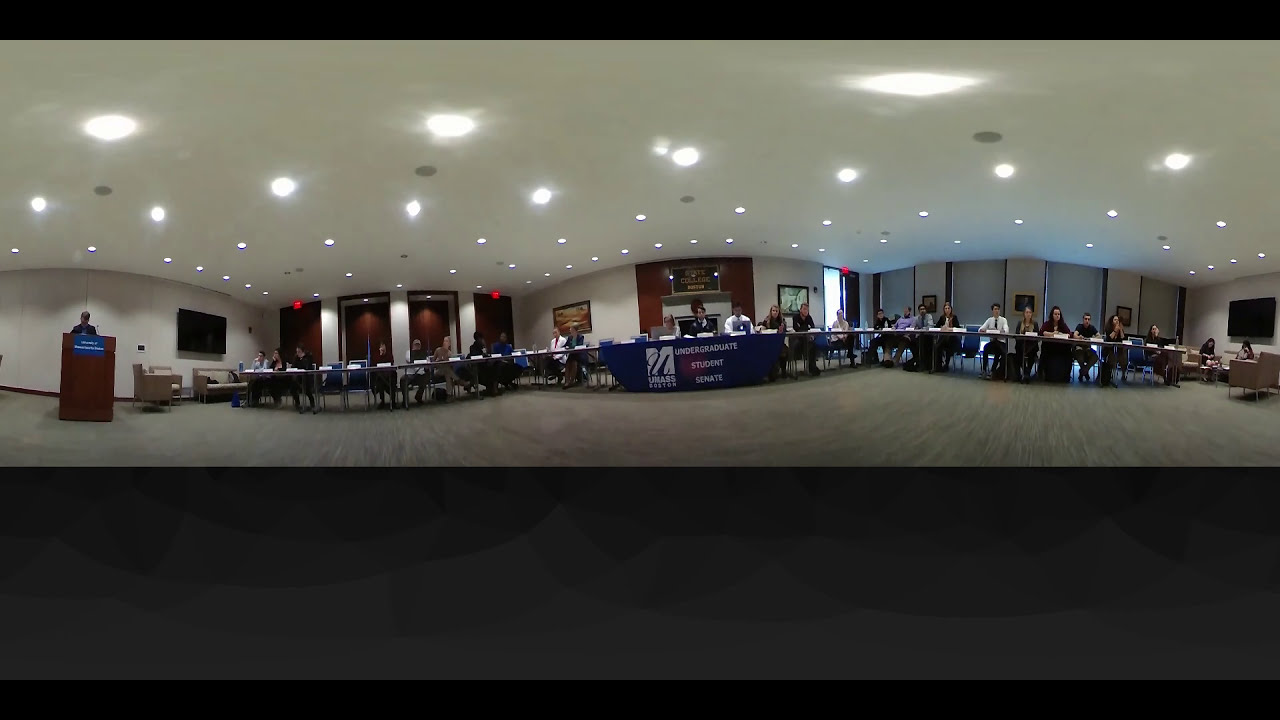The photo captures a 360-degree view of a large conference room with a gray carpet and white ceiling adorned with numerous recessed lights. Centered in the room is a long row of tables, side by side, draped in blue with the banner "Undergraduate Student Senate," marked by a white logo and text. The tables are arranged as if to face an audience, with multiple young males and females seated at them, each with a name placard. To the far left stands a wooden podium with a person speaking into a microphone. Against the back wall and right wall are modern office-type furniture and turned-off TVs, with two people seated on the furniture. The image appears slightly distorted, possibly due to being taken from a security or surveillance-type camera, and features thin black lines running horizontally along the top and bottom and a dark grey box occupying the bottom quarter of the image.